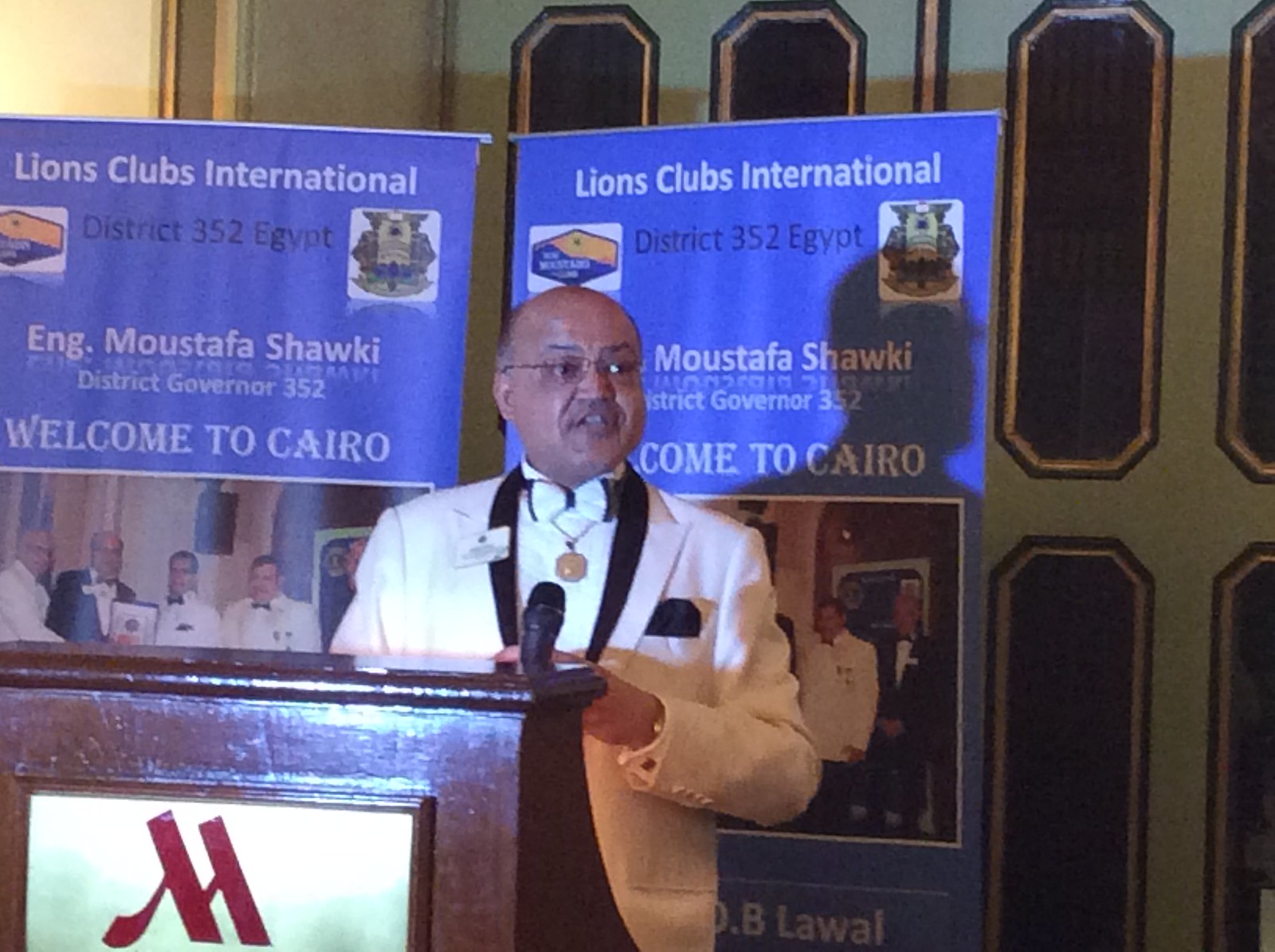In the image, a bald man with glasses stands behind a podium, appearing to be in the middle of making a speech. He’s dressed in a white tuxedo jacket with black lapels, a white and black bow tie, and wears a gold-colored necklace with a pink circle pendant. The podium, featuring a red "M" Marriott logo, supports a microphone in front of him. Behind him, two billboards display the text "Lions Clubs International District 352, Egypt" and "ENG Mustafa Shaki, District Governor 352, Welcome to Cairo." The setting is well-lit with natural light, providing a clear view of the scene.